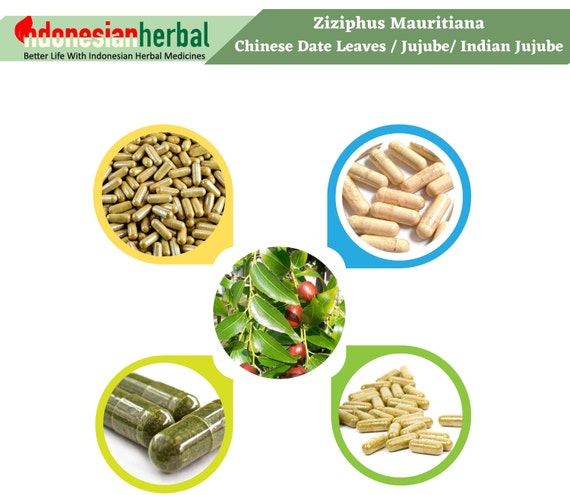The image showcases a collection of various capsules of Indonesian herbal medicines, organized around a central photograph of a plant with green leaves and red berries, possibly representing the jujube fruit. At the top left, a light green rectangle features the text "Indonesian Herbal" with "Indonesian" in red and white, and "Herbal" in lowercase green. Below in small black letters, it reads, "Better Life with Indonesian Herbal Medicines." To the right, a darker green rectangle lists the ingredients: "Ziziphus maritiana, Chinese date leaves, jujube, Indian jujube." Surrounding the central plant image are four smaller photos: the top left, highlighted in yellow, shows a heap of brown capsule pills; the top right, highlighted in blue, features a denser group of lighter brown capsules; the bottom left, outlined in lime green, depicts clear capsules with a green substance inside; and the bottom right, with a regular green highlight, displays more brown capsules. Each sub-image is framed with a semicircular cut-out towards the central plant photograph, illustrating the diverse forms of the herbal medicine capsules.